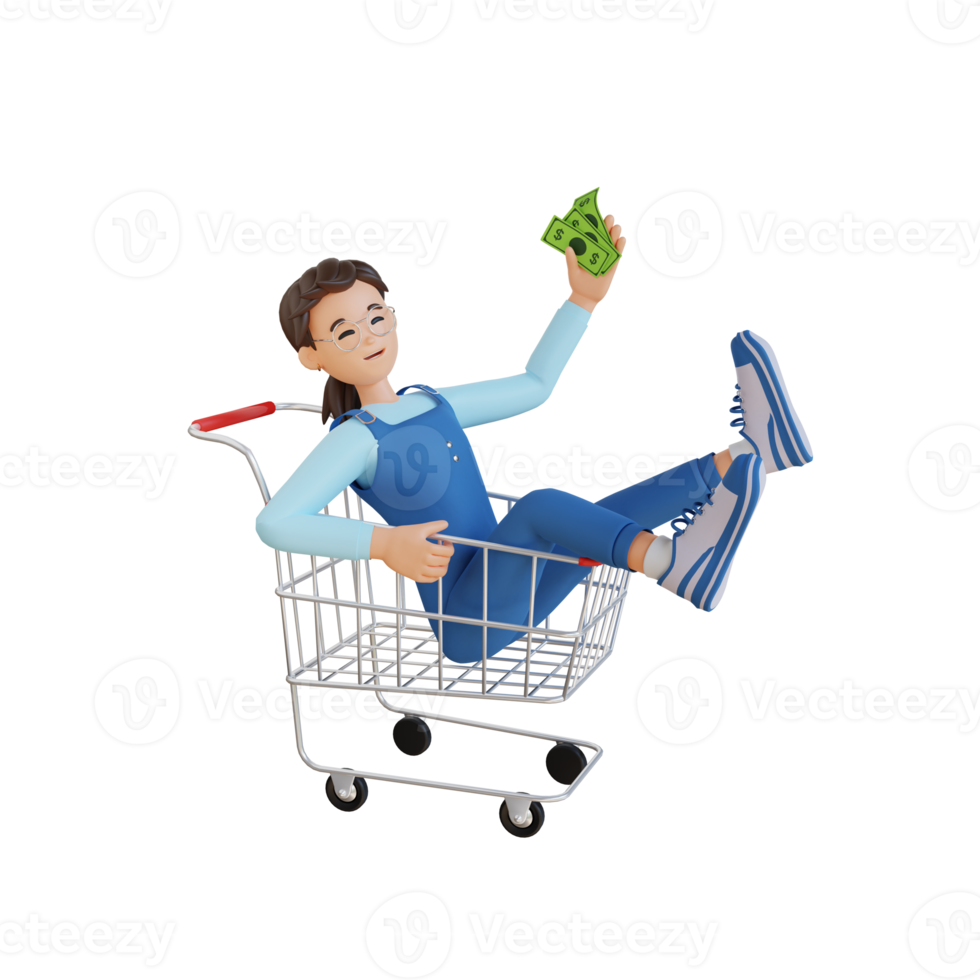The image is a detailed three-dimensional or cartoonish illustration of a young woman sitting inside a white, shiny metal shopping cart with black wheels and a red push handle. She is dressed in blue denim overalls with yellow buckles, a pale blue long-sleeved shirt underneath, and grey and blue sneakers with white socks. Her dark brown hair is tied back in a ponytail, and she wears grey-framed glasses with stick-figure eyes and a button nose, giving her a slightly animated expression. The woman, who appears Caucasian, is smiling subtly with lips appearing as a small slit. She is holding three green dollar bills in her left hand, raised cheerfully, and her right hand grips the side of the cart. Her bottom is seated firmly at the base of the cart with her legs hanging off the side, one leg raised in a carefree manner, embodying the spirit of a happy shopper.